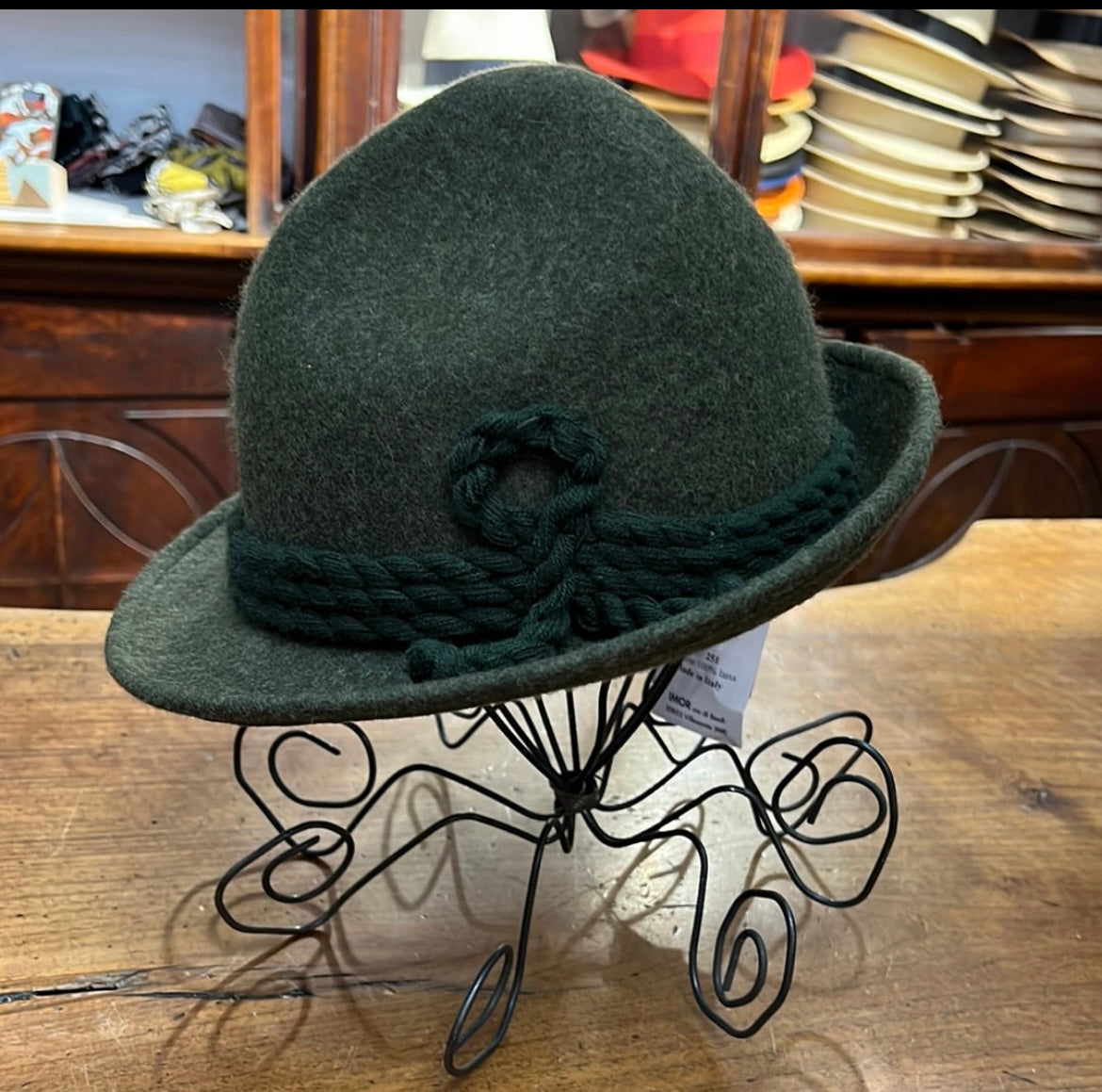This close-up product shot captures a black felt hat positioned prominently on a bent metal wire display, giving it an almost sculptural appearance with its four wiry legs. The hat features a tall, rounded top with a small brim, both constructed from the same black felt material. Accentuating the hat is a distinctive black braided rope running around the base of the crown, configured in three thick layers and looped into an intricate knot at the front. A tag hangs from the back of the hat, which rests on a light wooden table.

In the background, various other hats are visible, shelved neatly in a wooden display case. The assortment includes hats in white with black ribbons, colorful varieties, and cream-colored options with black ribbons. The room's ambiance is enriched by these diverse stacks of headwear, adding depth and interest to the overall scene. Hints of brown tones can be seen in the table and the background, contributing to a warm, inviting shop atmosphere.